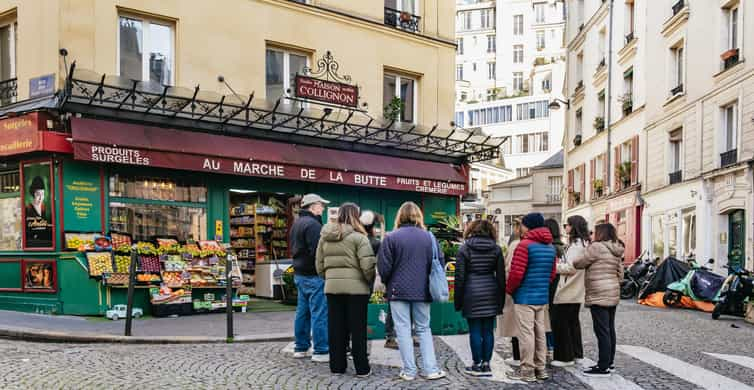The image depicts a bustling street corner in a European city, where a group of eight people, dressed in puffy jackets, are gathered in a semicircle around a store with a distinctive facade. The ground beneath their feet is cobblestone gray, and they appear to be in the middle of a crosswalk. The store front is a charming blend of colors: the first floor is green with a black awning, and above the awning, a cream-colored building facade with a red trim. The sign on the store reads "A.U. Marché de la Bouteille Fruits et Légumes," indicating it is a market selling fruits and vegetables. Displayed outside the store are various fruits in boxes, while a table with a blue tablecloth holds additional goods. Above the storefront, higher floors of the building have windows, suggesting residential apartments. To the right of the scene, more buildings in varying shades of tan and gray can be seen, along with a couple of parked motorcycles. Additionally, a banner with white writing reading "Mason Cullinan" is visible on one of the buildings. The overall scene is dynamic, capturing a moment of everyday life in what appears to be a quaint European locale.